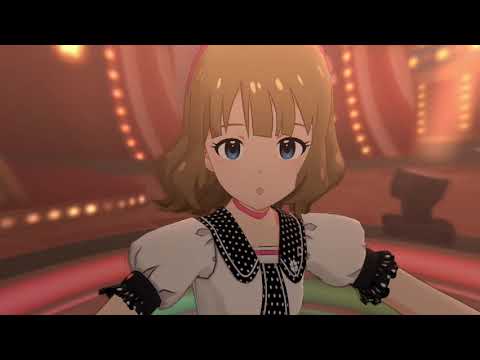The image depicts a digitally rendered, anime-style Caucasian girl centrally positioned and looking directly at the camera. She has strikingly large blue eyes, light brown shoulder-length hair with bangs, and a tiny mouth and nose, giving her a surprised expression. She's dressed in a white puffy shirt with polka dot accents on the collar and placard, complemented by black lacy cuffs on her sleeves. The scene in the background is blurry, featuring vibrant shades of pink, red, and yellow with hints of circular lights, giving an impression of a stage or game show setting. The background details are indistinct, enhancing the focus on the girl.